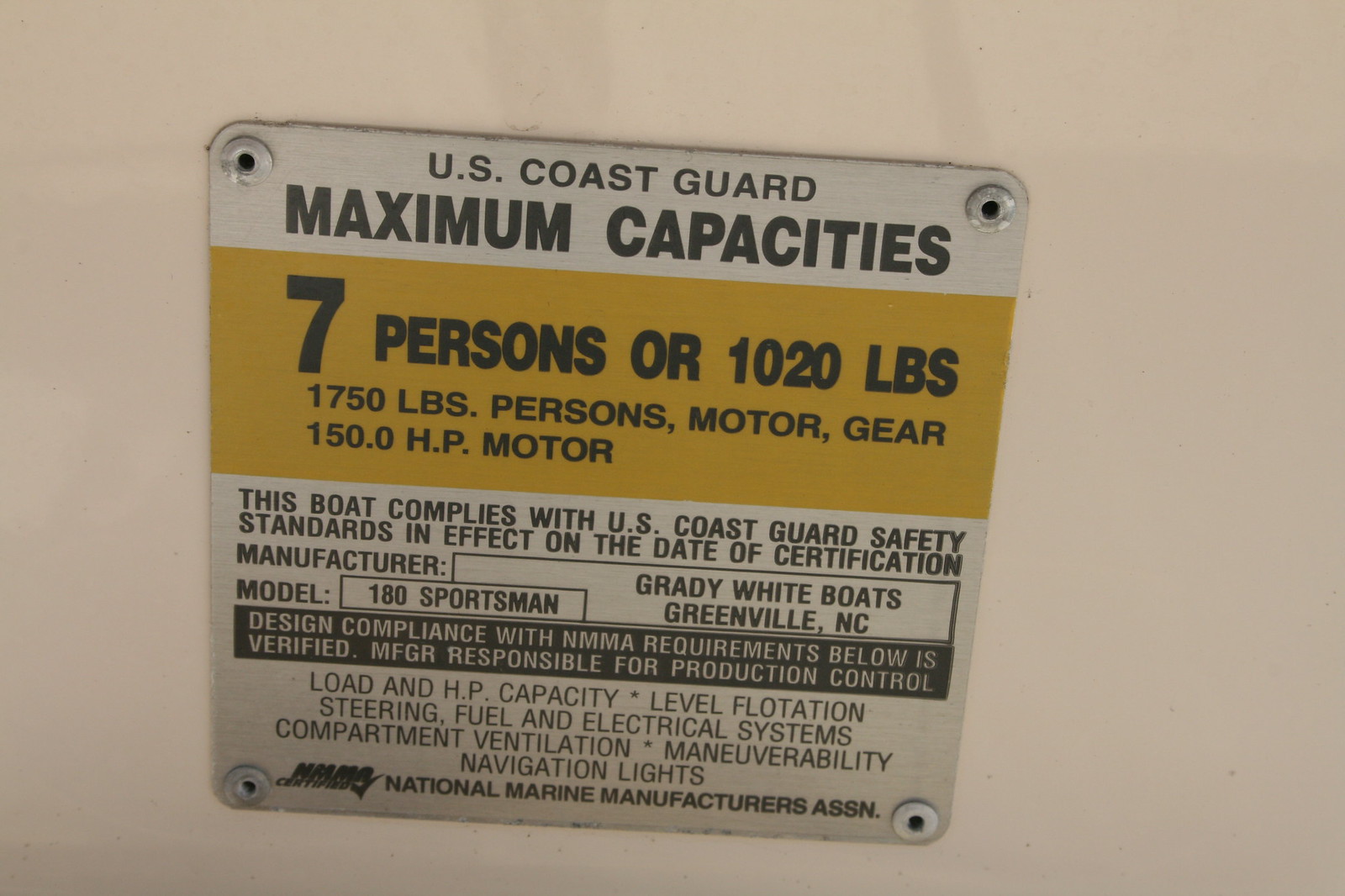The image shows a detailed U.S. Coast Guard warning label attached to a ship vessel. The metal label is mounted at an angle with four visible screws on a white surface, likely part of a boat. The label, which appears to be about 3 inches in size and has a rounded square shape, displays critical safety information in all capitalized text. The primary text, set in black against a white background and highlighted with a yellow rectangle, states: "U.S. Coast Guard Maximum Capacities, 7 Persons or 1,020 lbs, 1,750 lbs Persons, Motor, Gear, 150 HP Motor." Below this main section, smaller black font details additional compliance information within a black strip: "Design Compliance with NMMA Requirements Below is Verified. MFG are Responsible for Production Control." The text within the black strip is in white, further emphasizing compliance details. The warning label color scheme includes white, black, and yellow, serving as a clear and essential reminder of the vessel's capacity limits to ensure safe operation.